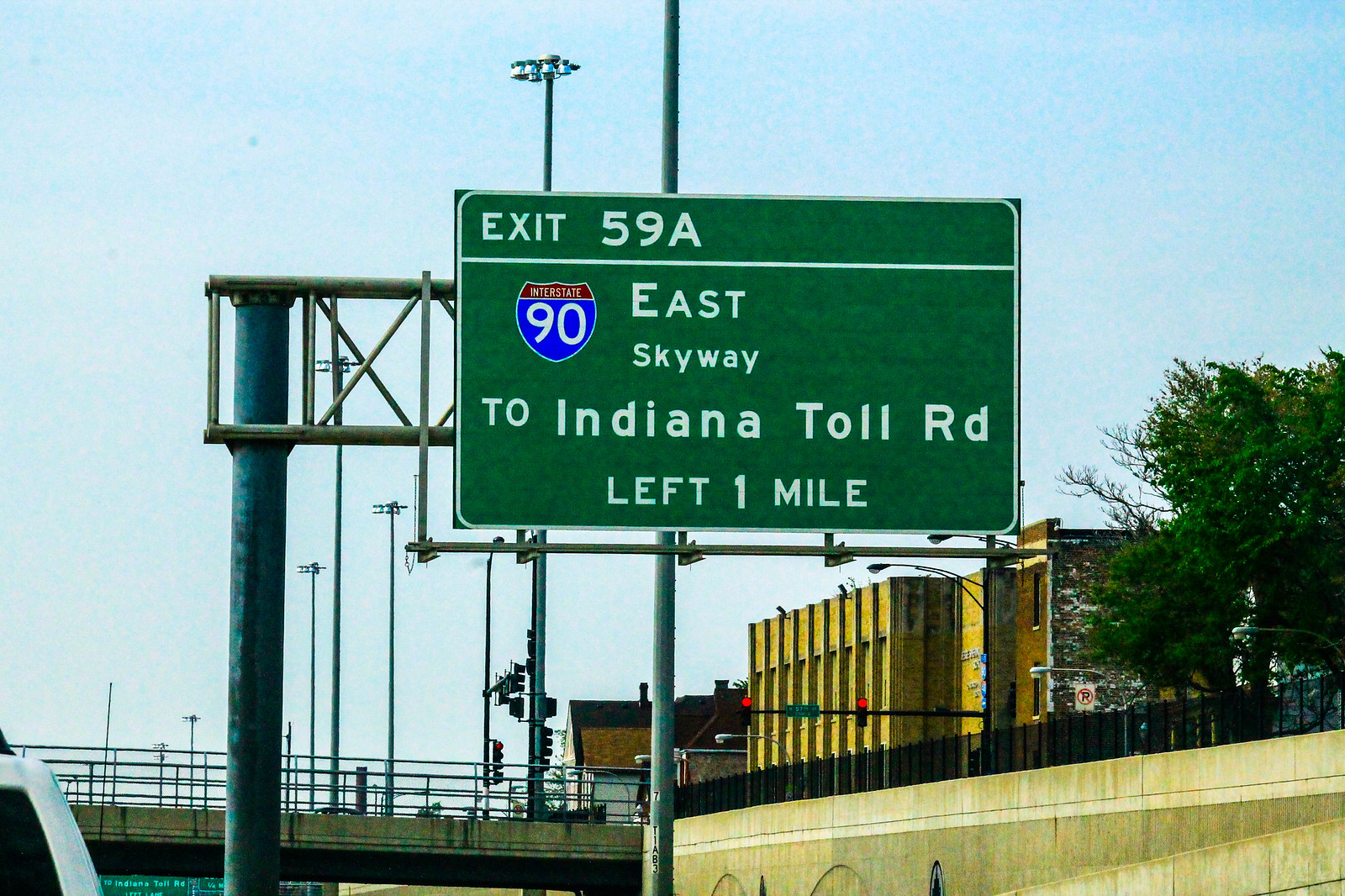This detailed photograph captures a bustling urban setting with a highway scene during daylight hours. Dominating the image is a large green highway sign with white lettering, mounted prominently on a sturdy metal pole above the roadway. The sign features the blue and red Interstate 90 shield and reads, "Exit 59A, Interstate 90, East Skyway to Indiana Toll Road, left 1 mile." Below the sign, a concrete barrier is visible, while further in the background, a bridge or overpass with metal railings spans the road. 

To the right of the sign, a vibrant green tree adds a touch of nature to the cityscape. The skyline includes a tall, aged yellow building adorned with pillars and situated near a cluster of utility poles and various traffic lights, all showing red signals at the moment. The sky overhead is mostly clear, providing a light blue backdrop that contrasts with the urban elements.

Additional details include a 'No Parking' sign visible on the building’s wall, a glimpse of the tops of vehicles on the overpass and likely the lower edge of a vehicle in the foreground. Colors in the image are primarily blue, white, green, and red, offering a vivid and realistic portrayal of city life intersecting with transportation infrastructure.